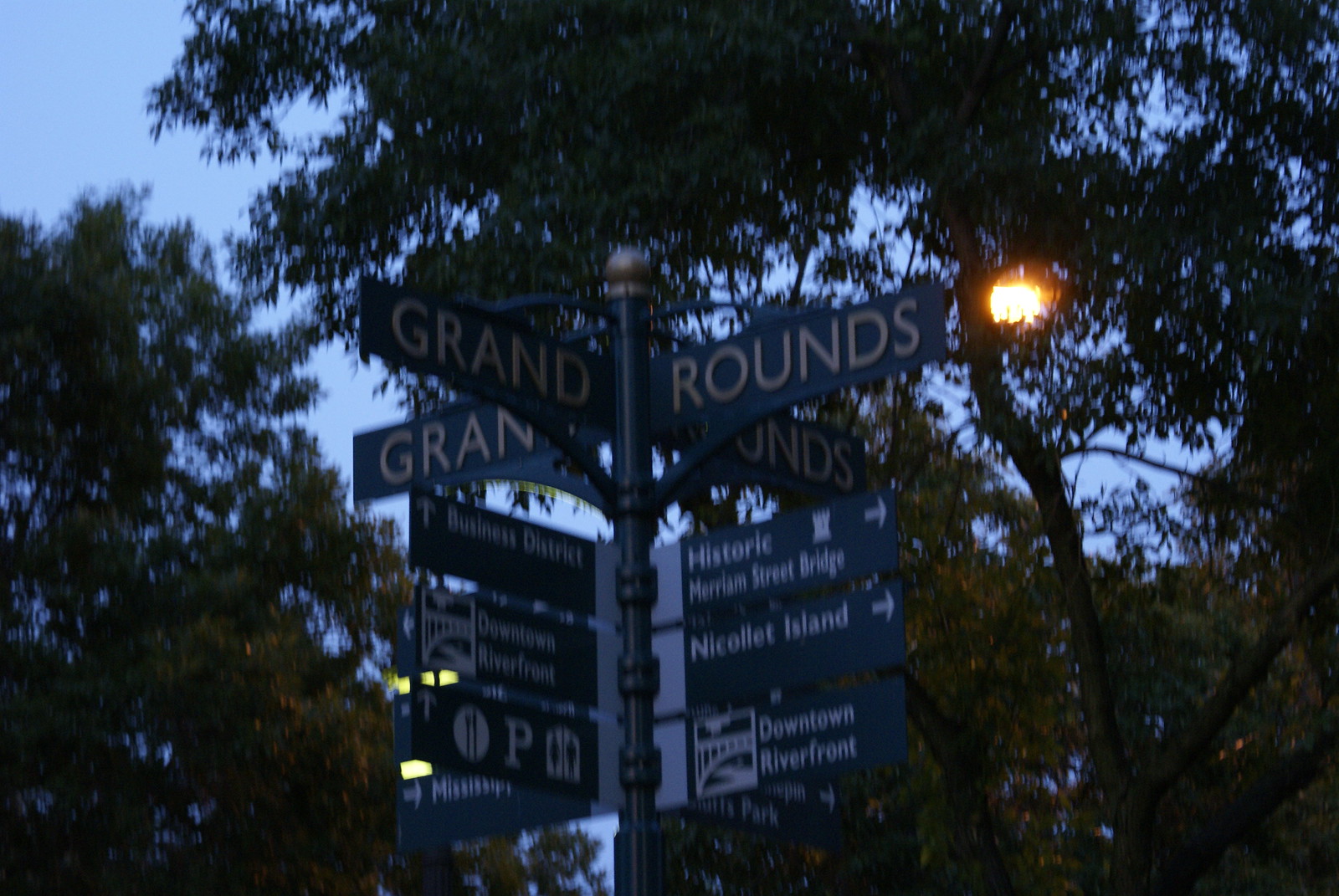In this evening photo captured at sunset, the darkening sky transitions into a light blue backdrop, softly illuminating the silhouetted tops and limbs of full trees. The scene centers on an ornate, black metal pole, intricately designed, supporting a four-way street sign. Each sign is crafted from matching black metal, adorned with bronze-colored lettering for a classic touch. Two pairs of signs bear identical street names, each set pointing in opposite directions. Below these primary signs, a cluster of additional directional signs guides pedestrians toward various local attractions, including the business district, the historic Merriam Street Bridge, Nicollet Island, and the Downtown Riverfront. The streetlights are already glowing warmly, casting a gentle light on the scene and enhancing the timeless charm of the setting.